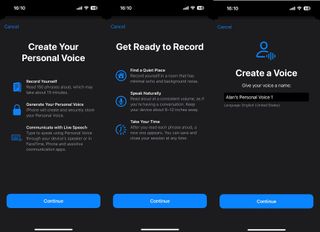In this screenshot, we observe a very small and blurred image primarily featuring a solid black background. At the top of the screen, the status bar icons are somewhat visible, including a battery icon, a partially discernible Wi-Fi icon, and a reception signal indicator represented by bars. Beneath these icons, there is a section with prominently large, bold white text. On the left side, the text reads "Create Your Personal Voice." To the right of this, there is instructions, "Get Ready to Record." Following further to the right, the text prompts, "Create a Video." Occupying the bottom portion of the screen, three blue action boxes are aligned horizontally, each containing the word "Continue" in white text inside the box, inviting the user to proceed with the available options.